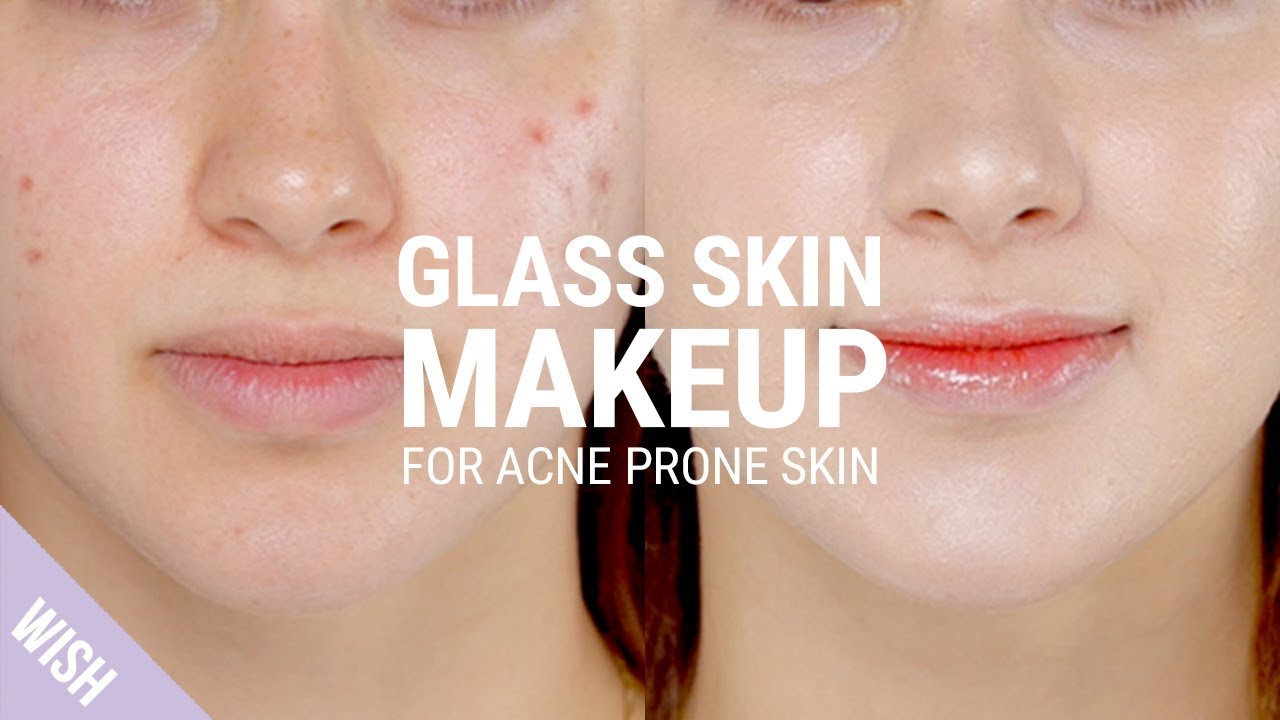The image is an advertisement for makeup, specifically designed for acne-prone skin, likely sold on Wish.com. It features a before-and-after comparison of the same Caucasian female's face from just below her eyes to slightly below her chin. On the left side, her face shows visible acne on both cheeks, dry lips, and hyperpigmentation along the nose and cheeks. Her hair appears to be a reddish-brown color. The right side displays her face with a clear complexion, indicating she is wearing makeup. Her skin has an opalescent sheen, and her lips are smooth with a pinkish-red tint, likely from chapstick or lip gloss. The central text across both halves reads "Glass Skin Makeup for Acne-Prone Skin," and a small purple triangle banner in the lower left corner says "Wish." The text is written in white, directly over the facial images, and there is no additional background.